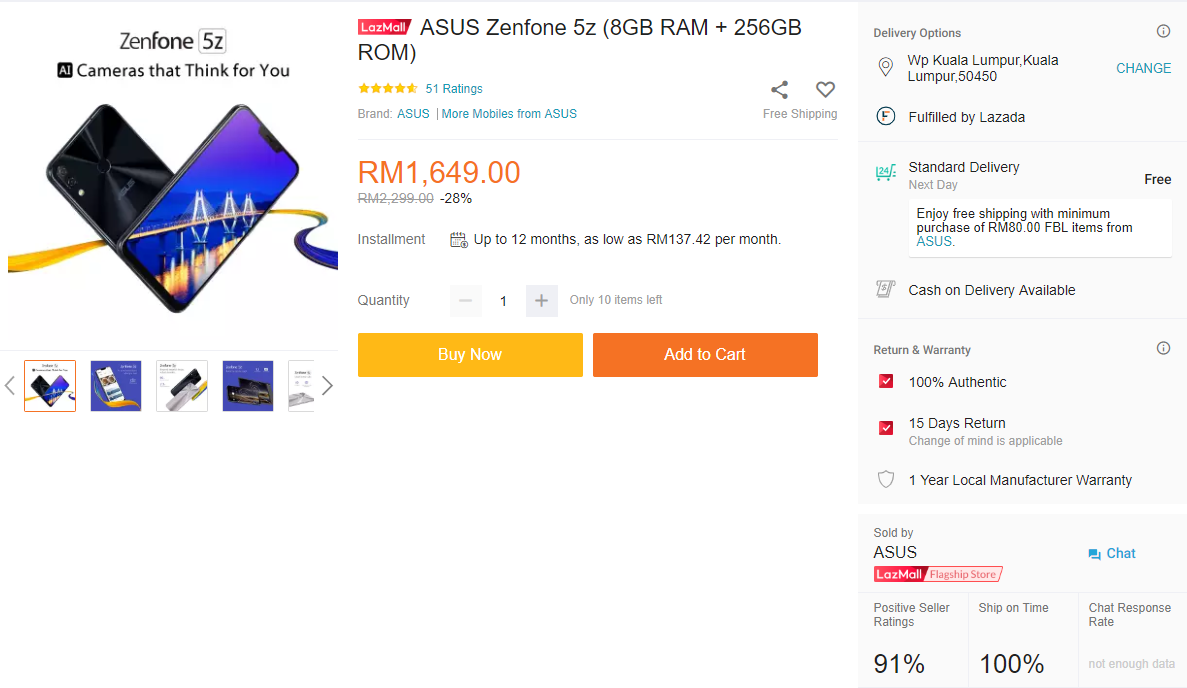This image depicts a detailed cell phone listing for the ASUS Zenfone 5Z. The layout of the listing is divided into three horizontal sections. 

On the leftmost section, the header reads "Zenfone 5Z" with the spelling "F-O-N-E". Below this, the tagline "Cameras that think for you" is displayed. A design element shows two intersecting smartphones; the left device has a black screen while the right one sports a blue screen adorned with a curved yellow and blue line. Further down, there are five images showcasing the ASUS Zenfone 5Z.

The middle section features the product name "ASUS Zenfone 5Z" accompanied by 51 ratings, indicating an average of nearly five stars. Below this, the brand name "ASUS" is highlighted. To the right of the brand name text, icons for free shipping, sharing, and favoriting the item are presented. The price is prominently displayed in orange as RM 1,649.00, with an additional note indicating that the phone can be purchased with a payment plan of up to 12 months at RM 137.42 per month. The purchasing options are clearly marked with a yellow "Buy Now" button on the left and an orange "Add to Cart" button on the right.

The rightmost section has a light gray background and includes information on delivery options, the fulfillment address by Lazada, and various return and shipping details.

Overall, this image provides a comprehensive visual summary of the ASUS Zenfone 5Z listing, complete with product visuals, pricing, and purchasing details.